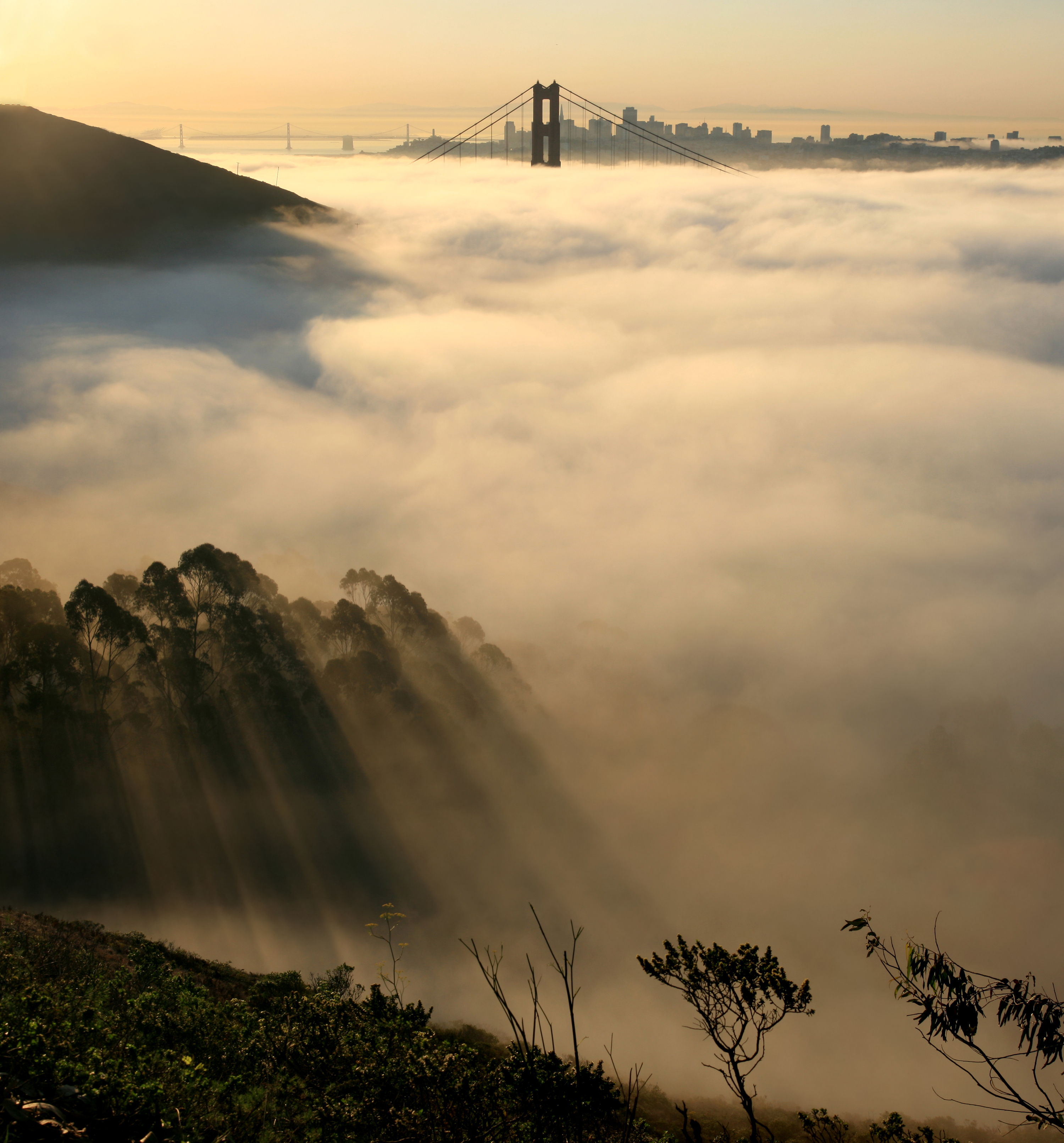This captivating image features a bridge reminiscent of San Francisco's iconic Golden Gate Bridge, draped in a dense blanket of fog. While the bridge's identity remains uncertain, its towering support structures and suspension cables emerge starkly above the thick mist, which obscures the roadway below. The fog, resembling cotton clouds, creates an ethereal atmosphere as it envelops the water, making the bridge seem as though it floats on a sea of puffy whiteness under the sunlight.

In the backdrop, a silhouette of a distant city peaks through the fog, accompanied by another, more straightforward bridge. This secondary bridge, likely a car thoroughfare, contrasts with the grandeur of the primary bridge by its simpler design. The coastline closest to the camera is defined by rocky bluffs jutting dramatically into the fog, with patches of grass and scattered small trees adding a touch of green to the otherwise monochromatic scene.

The sun illuminates the fog, giving it a bright, cloud-like appearance and enhancing the surreal, breathtaking quality of the landscape, making it a captivating image of nature intertwining with urban architecture.